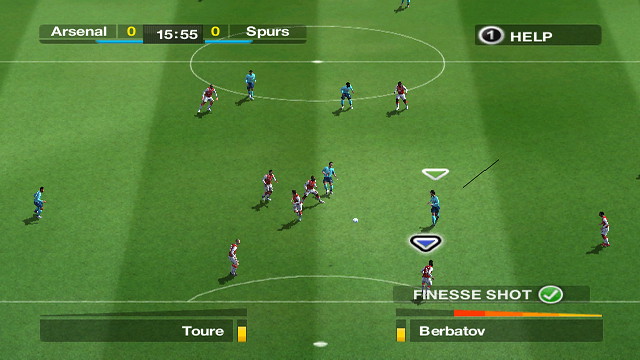A detailed caption for the described image could be:

"In the virtual soccer game displayed on screen, players are positioned on a lush, green soccer field. Notable features include two large white circles, one near the front and one towards the back of the field, each intersected by a white line running through their centers. A distinctive triangle hovers above the heads of two specific players, indicating active control. The player in the blue uniform faces off against another in a red and white uniform, creating a vivid contrast. At the bottom left corner of the screen, text reads 'Touré,' while the bottom right corner displays 'Berbatov.' Above Berbatov's name is a progress bar that transitions from a yellow shade to red as it fills, currently almost full with the left side unfilled. The top left corner provides match details, showing 'Arsenal 0, 15:55,' indicating the game timer, followed by '0 Spurs,' highlighting the ongoing score with 'Arsenal,' currently holding no goals against 'Spurs,' also goalless. The image captures a tense moment in an animated soccer match, brimming with competitive energy."